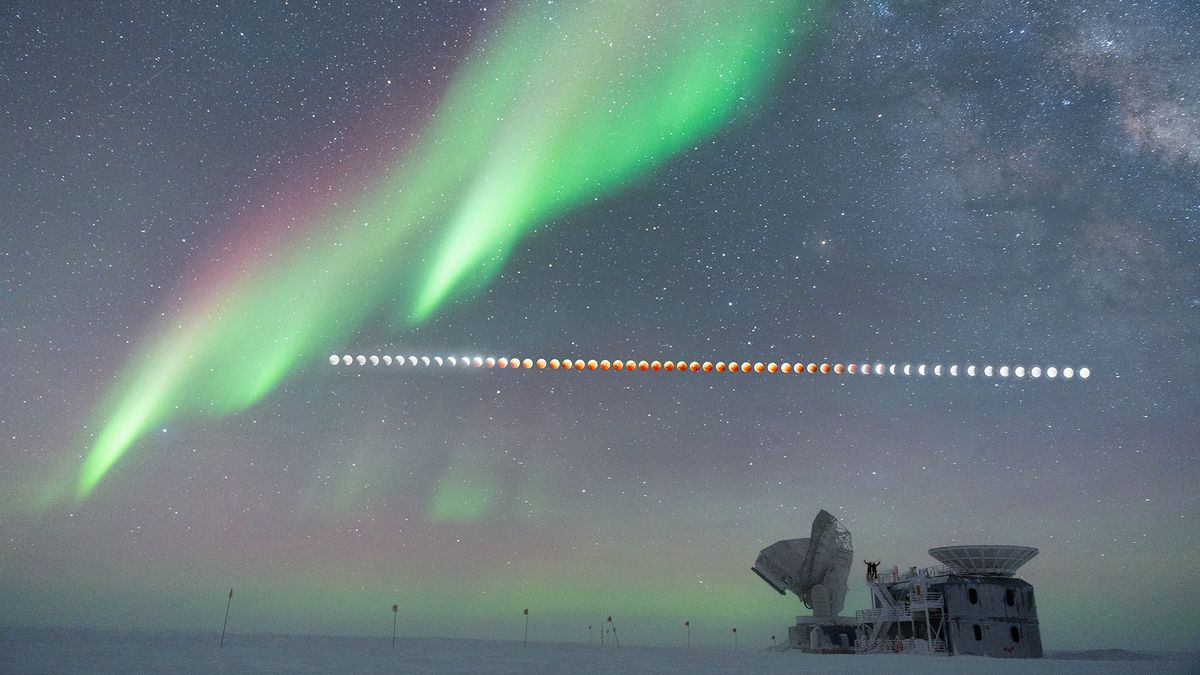The photograph captures a breathtaking twilight scene, likely set in a remote, snowy location such as Alaska or Antarctica, beneath a clear, star-studded sky. Dominating the sky is a mesmerizing display of the northern lights. This aurora starts as a reddish-pink hue at the top and transitions into vibrant neon green and white, forming a wispy arc across the sky. 

Beneath this ethereal light show, a sequence of moons in various phases stretches across the center of the image, possibly the result of a time-lapse photography capturing a lunar eclipse. The moons display a gradient of colors, transitioning from bright white to an orange-brown hue and back to white, indicating the shadow's movement across their surface.

On the snow-covered ground below, a large observatory or research station is visible. This structure, resembling those found in polar research facilities, has several attached instruments that appear to be telescopes or satellites for celestial observation. Two people are seen standing on top of the building at the edge of a staircase, arms raised, seemingly reveling in the celestial spectacle above. The combination of the aurora, the phases of the moon, and the distant nebula on the right side of the image creates a scene of natural wonder and scientific exploration.